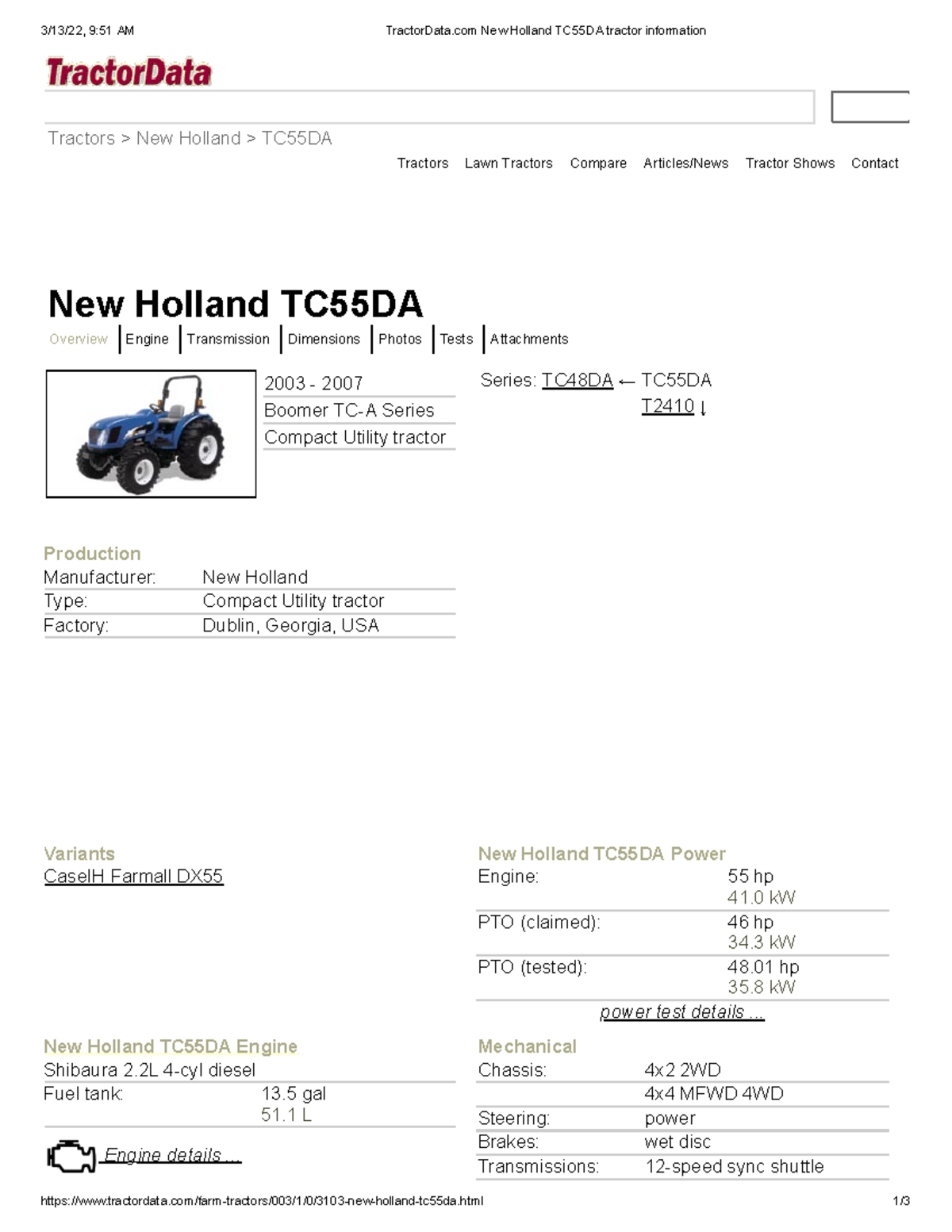The image appears to be a detailed specification sheet or a web page dedicated to the New Holland TC 55 DA tractor. At the top, the title "Tractor Data" is prominently displayed in red. Directly beneath it, the heading "New Holland TC 55 DA" is shown in bold text. Underneath this heading is an image of a blue tractor labeled "New Holland TC 55 DA," which was produced from 2003 to 2007 as part of the Boomer TCA series of compact utility tractors.

Further details include the manufacturer and type of the tractor: it is a New Holland compact utility tractor, manufactured in Dublin, Georgia, USA. The sheet also breaks down various specifications:

- **Variances:** It lists different series such as K Castle H and New Holland TC 55 DA.
- **Power:** 
  - Engine: 55 HP (41.0 kilowatts)
  - PTO Claimed: 46 HP (34.3 kilowatts)
  - PTO Tested: 48.01 HP (35.8 kilowatts)

The specifications cover powertrain and mechanical details:
- **Chassis:** Options include 4x2 2WD and 4x4 MFWD 4WD.
- **Steering:** Power steering.
- **Brakes:** Wet disc brakes.
- **Transmission:** 12-speed sync shuttle.

To the left of the image is a smaller picture showing the engine. Below it are engine specifics:
- **Engine Type:** Shibara
- **Displacement:** 2.2 L four-cylinder diesel
- **Fuel Tank Capacity:** 13.5 gallons (51.1 liters)

Overall, this detailed sheet provides comprehensive information about the New Holland TC 55 DA tractor, encapsulating its production history, power specifications, mechanical features, and engine details.